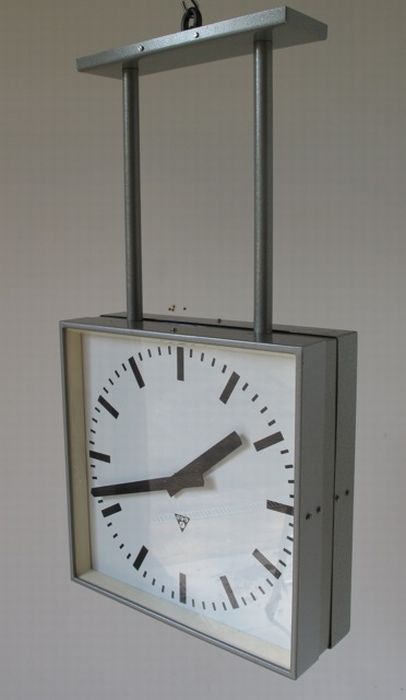A close-up photograph of a uniquely designed clock displayed on a stand. The clock itself is crafted from stainless steel and is suspended upside down from a small metal hook attached to its top. The stand features a flat, rectangular stainless steel base from which two sleek metal bars extend upwards to support the clock. The clock's square frame is also composed of stainless steel, and it showcases a minimalist white face. The time is indicated by bold black minute and hour hands, which move along without traditional numerals. Instead, thick black stripes denote the hour markers, with four thinner black stripes positioned between each hour to mark the minutes. Notably, an inverted triangle sits beneath the clock hands, adding an artistic flourish to this modern timepiece design.